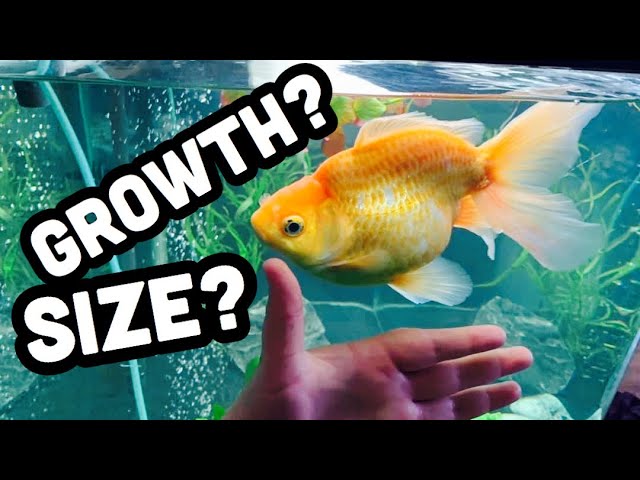The image, clearly a thumbnail likely for a video, features a massive goldfish inside a tank. The goldfish exhibits a striking gradient of orange and yellow, with more orange on the top, transitioning to a pale yellow near its pronounced belly. Its fins also display this color gradient, ending in pale yellow to white tips. The fish is swimming against a backdrop of green plants, creating a rich contrast with the bluish tone of the water. A left hand, colored in purple and pink hues, is positioned below the fish with the thumb raised and fingers extended towards the right, serving as a size comparison to emphasize the fish's enormous scale. Additionally, a blue hose is visible running through the tank, suggestive of the aquarium's filtration system. The image is framed by thick black letterboxing at the top and bottom, which enhances its video-thumbnail appearance. On the left side of the image, large white text with a black outline states "Growth?" and "Size?", hinting at the astonishing size of the goldfish. The combined elements emphasize the goldfish's impressive proportions and the curious context intended by the text.